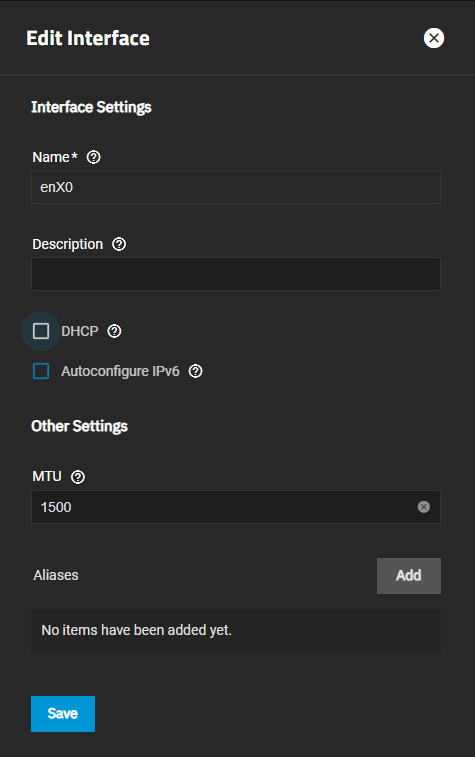The image features a user interface for editing network settings, displayed against a black background. At the top left corner, white text reads "Edit Interface," and on the top right corner, there is a white "X" close button. 

Below this header, a column of text along the left side includes the label "Interface Settings." The first setting is named "Name" with an asterisk indicating it is a required field. Adjacent to this label is a text box containing the text "enxo." 

Further down is a label for "Description," paired with an empty text box. Following this, there are two checkbox options: "DHCP," which is unchecked, and "Auto Configure IPv6," which is also unchecked but highlighted in blue. 

Beneath these checkboxes, the label "Other Settings" is shown, with a subsection for "MTU" that includes a text box containing the value "1500."

The next section is labeled "Aliases." To the right of this label, there is a gray button with white text that reads "Add." Just below it is another text box with white text stating "No items have been added yet."

Finally, at the bottom left corner of the interface is a blue rectangular button with white text that reads "Save."